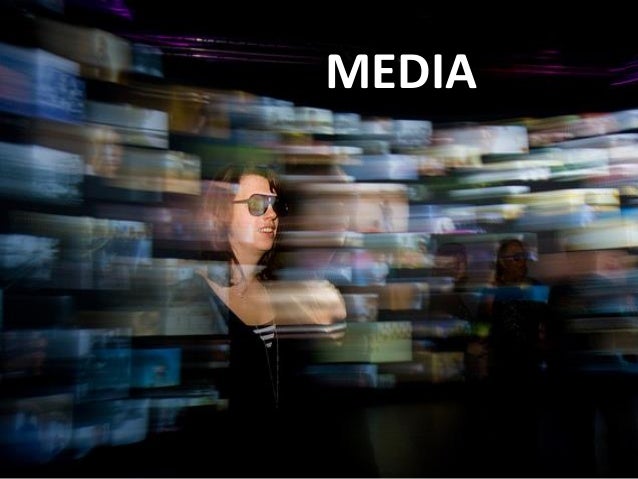The image features a black background with the word "MEDIA" prominently displayed at the top in large, white, all-capital letters. Below this, a horizontal purple stripe extends across the width of the image, framing the word without intersecting it. The central part of the image is a chaotic collage of blurry, rectangular prisms, reminiscent of multiple TV screens flashing rapidly and blending together. Among these prisms, several faces emerge, but the most distinct is that of a woman with brown hair and black sunglasses, smiling with her teeth showing. She wears a black dress with white and black stripes in the v-neck area. Another face, possibly of another woman with similar black sunglasses and long hair, appears on the right side. The overall effect is a dynamic and disorienting mixture of visuals, heavily emphasizing the theme of media saturation.